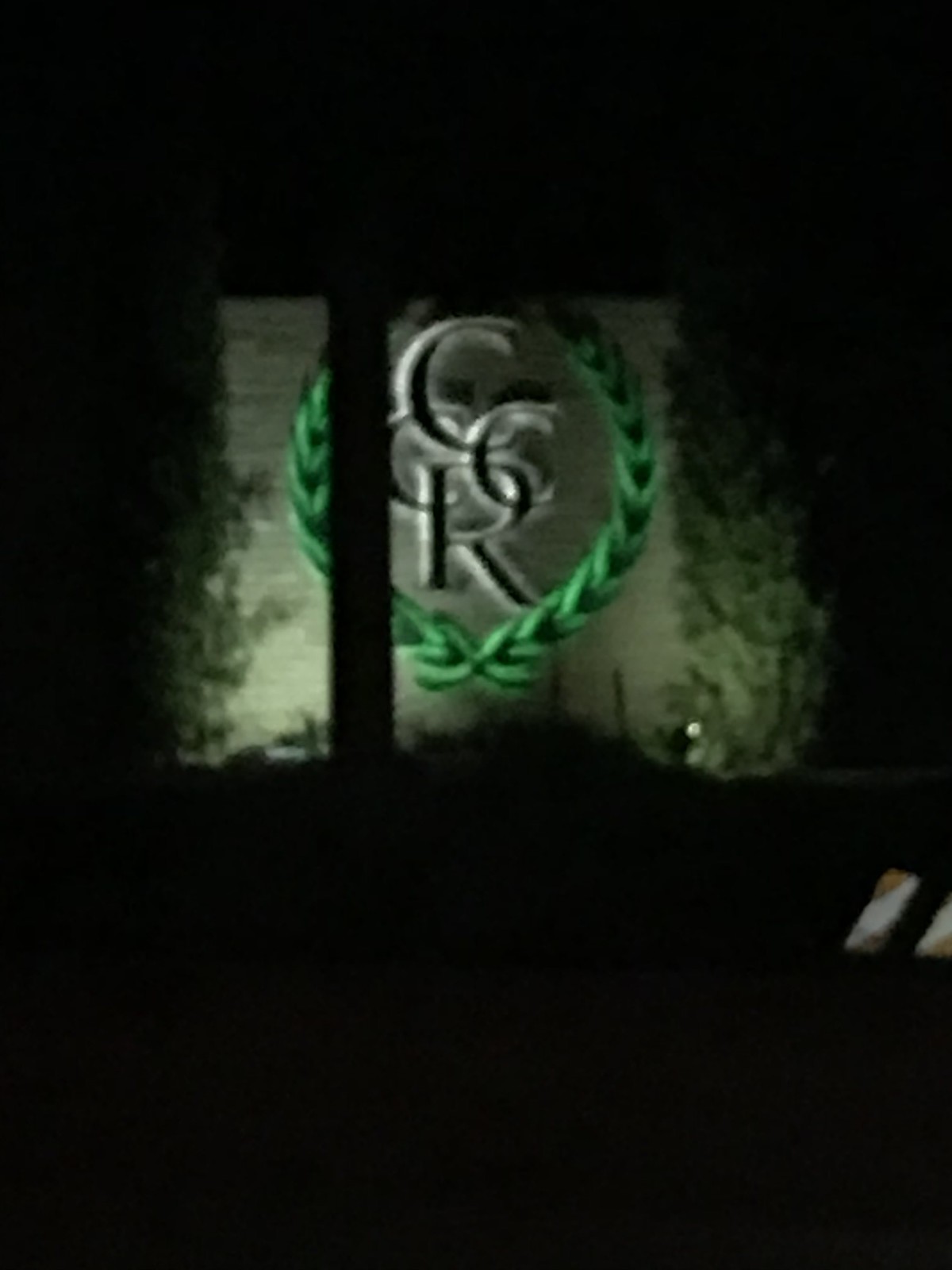Illuminated against the pitch black of night, a stone sign commands attention. The sign, likely belonging to a hotel or an apartment building, features overlapping letters arranged vertically: a single "C" at the top, two "C"s in the middle, and an "R" at the bottom. Encircling the entwined letters is a lush green wreath, reminiscent of Olympic laurel crowns. Ivy and foliage frame the sign on both sides, adding to the organic charm. The scene is only made visible by strategically placed lights at the base of the sign, which accentuate the stone texture and partially lit greenery, while the rest of the environment remains shrouded in darkness.